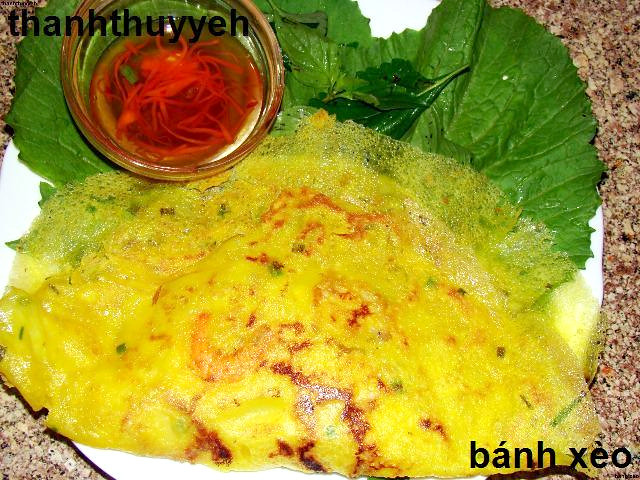The image features a traditional Vietnamese dish known as Bánh Xèo, which is a savory Vietnamese pancake that closely resembles a delicate, thin crepe or omelette. The yellow pancake is filled with what appears to be shrimp and assorted herbs, and its edges are thin and semi-transparent, indicating it was likely cooked in a wok. The Bánh Xèo is presented on a white plate, resting on a bed of large green lettuce leaves, adding to its visual appeal.

In the upper left corner of the image, black lettering spells "Phan Thuy," while the bottom right corner has "Bánh Xèo" also in black letters. Accompanying the dish is a small, clear ramekin filled with what looks like a traditional dipping sauce, containing either shredded carrots or daikon radish, and possibly red chilies, enhancing the dish's authentic flavor profile. The backdrop of the table appears to be made of a beige, brown, and tan marble or granite, adding an elegant touch to the presentation.